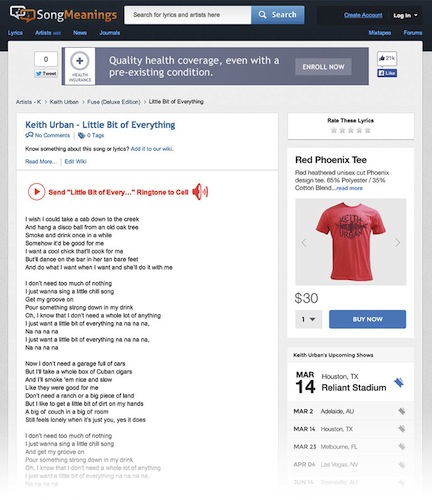**Detailed Caption:**

The central focus of the webpage is the Song Meanings website, featuring its distinctive logo—two speech bubbles, each containing a music note. To the right of the logo is a search bar prompting users with "Search for lyrics and artists here," and adjacent to it, buttons for "Create an Account" and "Login" are prominently displayed.

Navigation tabs are situated just below these elements, offering links to various sections such as Lyrics, Artists, News, and Journals. Below this navigation bar, an advertisement for health insurance captures some screen real estate.

Further down, the featured content centers around the song "A Little Bit of Everything" by Keith Urban. This section includes an audio player for listening to the track and an option to send the ringtone to a call. The complete lyrics for the song are presented, with a rating system to the right, allowing users to rate the lyrics from zero to five stars.

Additionally, to the side of the lyrics, there's a promotion for a Red Phoenix t-shirt, priced at $30. However, the details on this promotional item are somewhat obscured due to small text size. Overall, the webpage is dedicated to providing users with not just song meanings and lyrics but also various interactive and commercial elements.